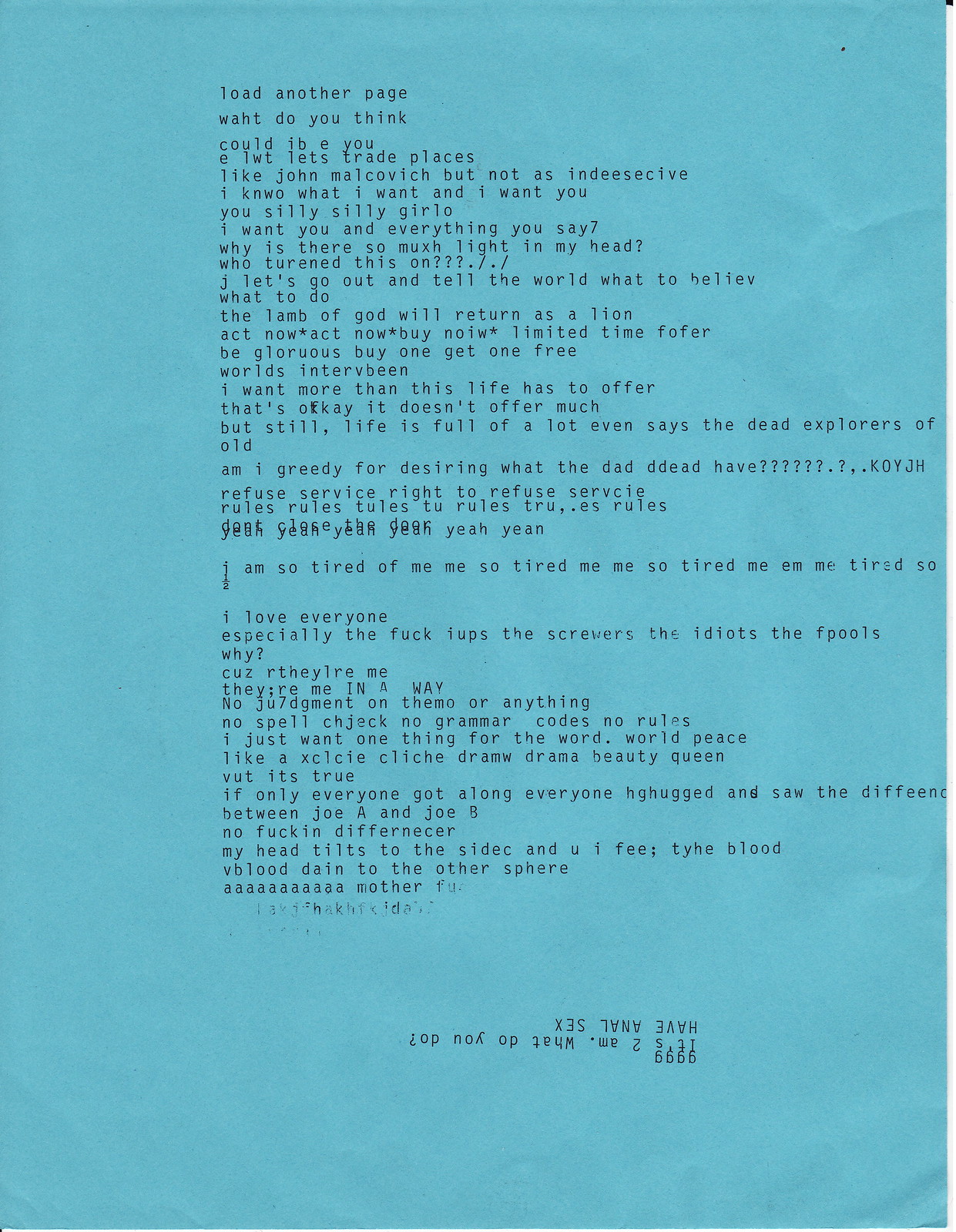The image is of a rectangular, blue piece of paper resembling a robin's egg or Tiffany blue. It appears to have been typewritten and contains several paragraphs of text, marked by numerous spelling and grammatical errors. The top of the document starts with the phrase, "load another page," followed by a mixture of coherent and jumbled sentences. Notable lines include, "What do you think? Could I be you? Let's trade places, like John Malkovich but not as indecisive. I know what I want, and I want you, you silly silly girl-o. I want you and everything you say. Why is there so much light in my head? Who turned this on?" 

There are random sequences of letters and numbers scattered throughout, and some text is over-typed, which suggests the typewriter ribbon might have been stuck. The document also features additional lines of print at the bottom, printed upside down as if the paper were re-inserted incorrectly into the typewriter. Phrases like "act now, act now, buy now, limited time offer, be glorious, buy one get one free," appear, adding to the overall cryptic and nonsensical nature of the content.